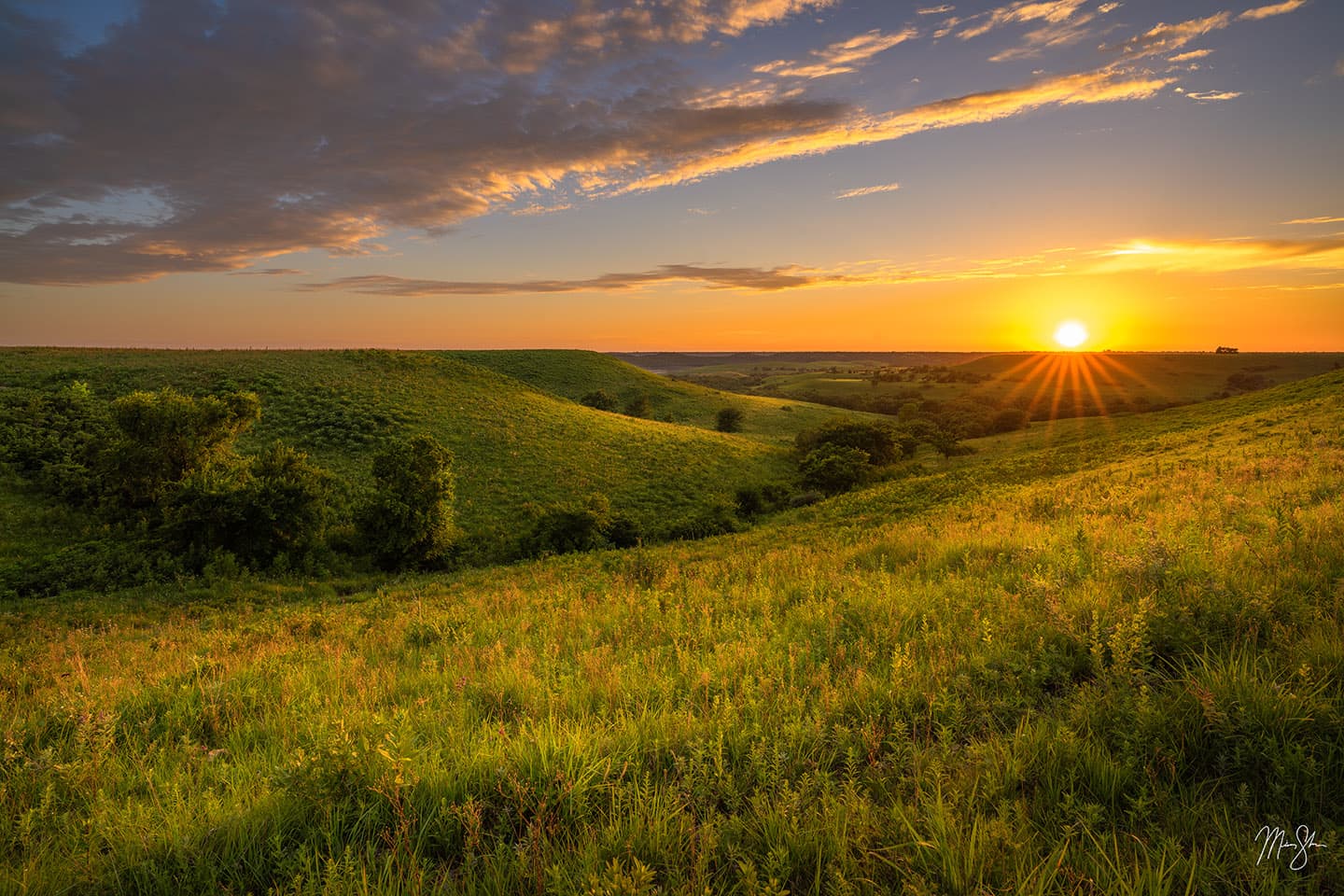This image captures the serene beauty of a grassy field during sunrise or sunset. The foreground is dominated by a lush meadow with interspersed weeds and bushes, giving it a brushy appearance. These plants create a reddish-gold tint amidst the green grasses. The field stretches toward the horizon, where a body of water with a subtle blue tint lies. The sky transitions from a deep blue at the top to a warm orange near the horizon, with the sun prominently glowing yellow on the right side of the image. Its orange rays bathe the landscape in a golden glow. The sky on the right is predominantly orange, fading to blue as it rises. On the left, the sky features a gradient from pinkish hues near the horizon to blue above, dotted with gray clouds partially illuminated in golden light. This harmonious blend of colors and natural elements captures the tranquil essence of the scene.